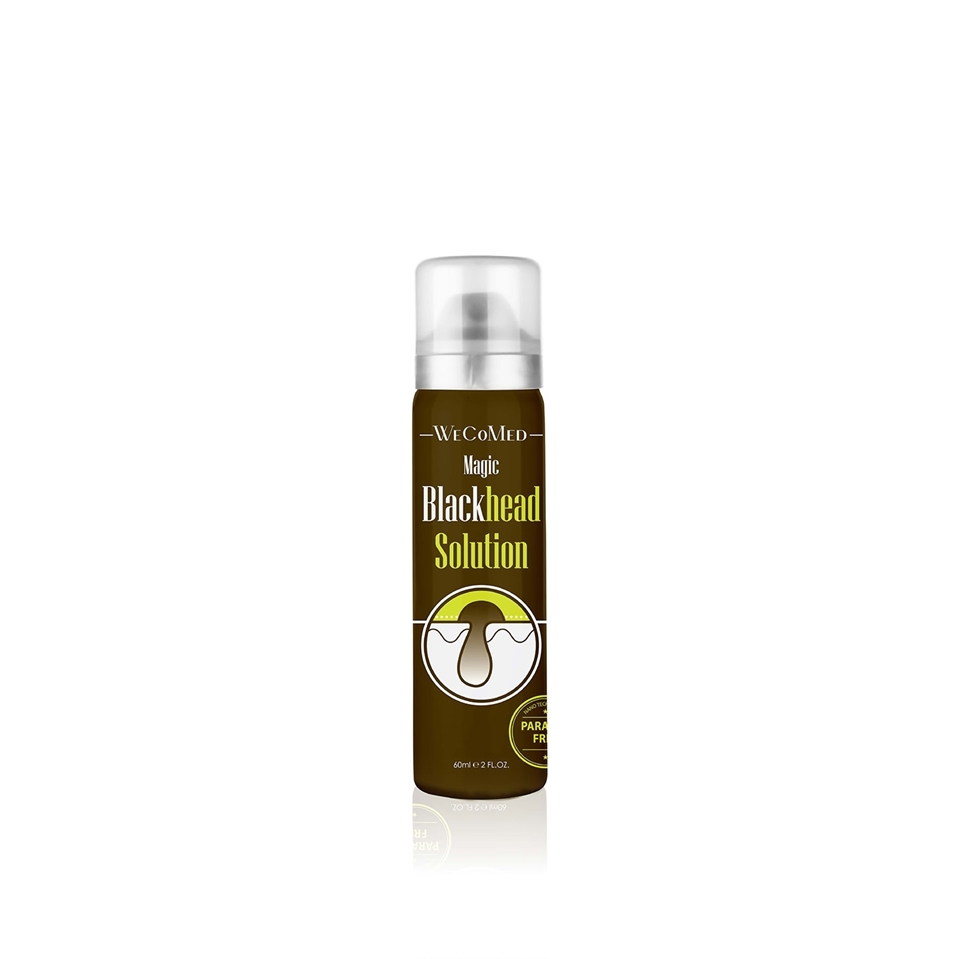This vertical image depicts a 60ml (2 fl oz) bottle of "Magic Blackhead Solution" by WeCoMed, designed for treating blackheads. The bottle itself is dark brown with white and yellow printing, and features a removable clear cap. At the top, the brand name "WeCoMed" appears in white lettering, followed by the product name "Magic Blackhead Solution". The word "Magic" is in smaller white font, while "Blackhead" is rendered with "Black" in white and "head" in yellow. The word "Solution" is entirely in yellow. Additionally, the bottle highlights that it is paraben-free, although this label is partially cut off in the image. Below the product name, there is an illustration showing the anatomy of a blackhead both above and beneath the skin, with the skin depicted in white and the blackhead set against a greenish-yellow background. The bottle also has a mirror image effect that fades toward the bottom.